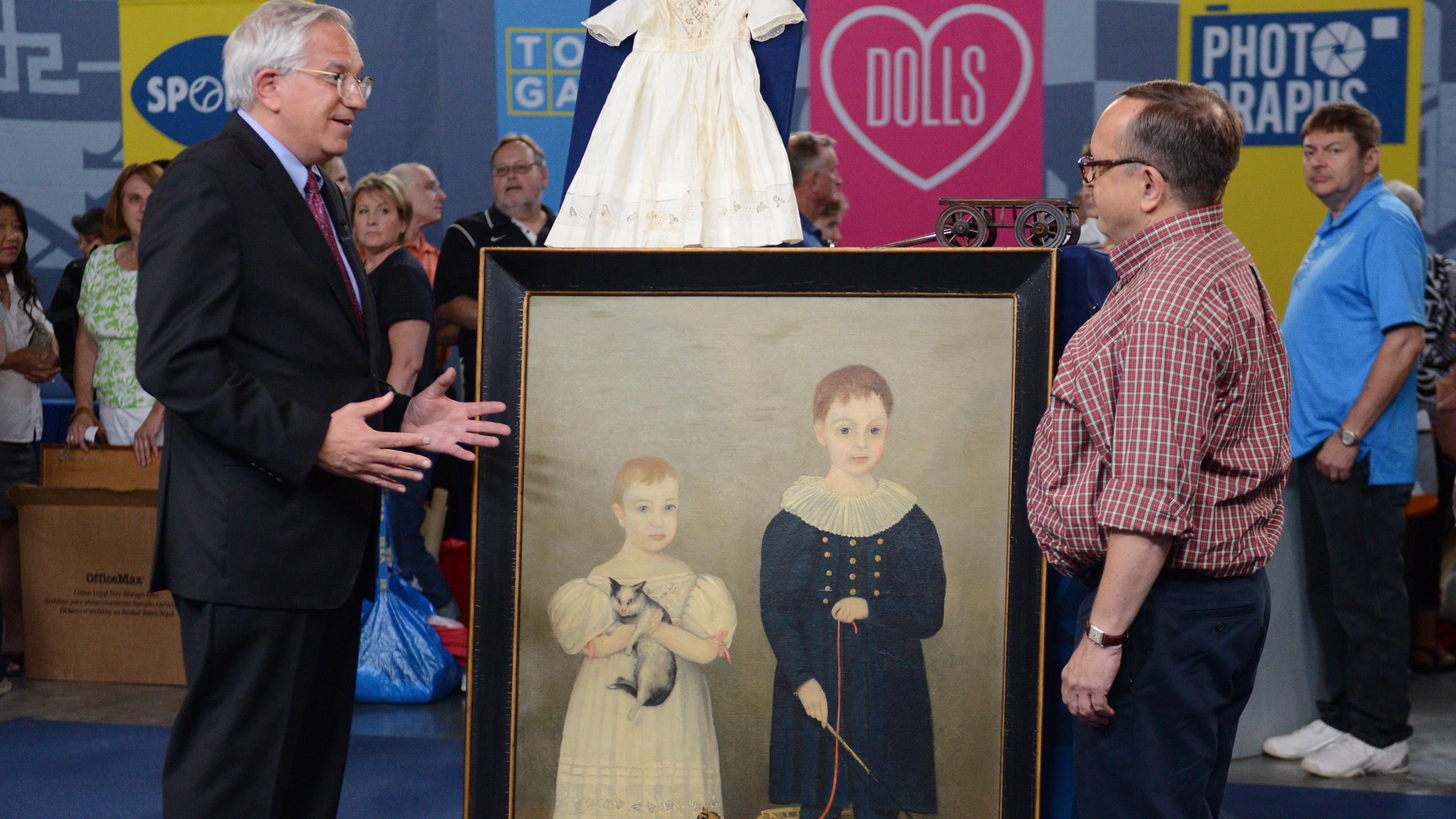This color photograph appears to be a scene from the television show "Antiques Roadshow," typically aired on PBS. The focal point of the image is two men engaged in a conversation, presumably an appraiser and an owner discussing a valuable item. On the left, there is an older gentleman with white hair, clad in a black suit, white collared shirt, red necktie, black pants, and wearing glasses. He is facing to the right, hands extended as if explaining something. Next to him stands a younger, heavier man with brown hair and glasses, dressed in a red and white t-shirt and blue trousers with the sleeves of his plaid shirt rolled up. Between them is an antique oil painting, framed in elegant gold and black. The painting portrays two children, likely from the 16th to 18th centuries. The taller child, possibly a boy about eight years old, wears a long-sleeved blue dress with brass buttons and a ruffled collar, and holds a red string extending off the canvas. The smaller child, potentially around five, is in a white dress with puffy sleeves, holding a black and white cat. The backdrop reveals a bustling scene with people lined up, some carrying items, indicative of a typical appraisal setting. There are visible signs including one with the word "Dolls" in pink along with a heart, and another saying "Photographics" against a blue background with a yellow border.